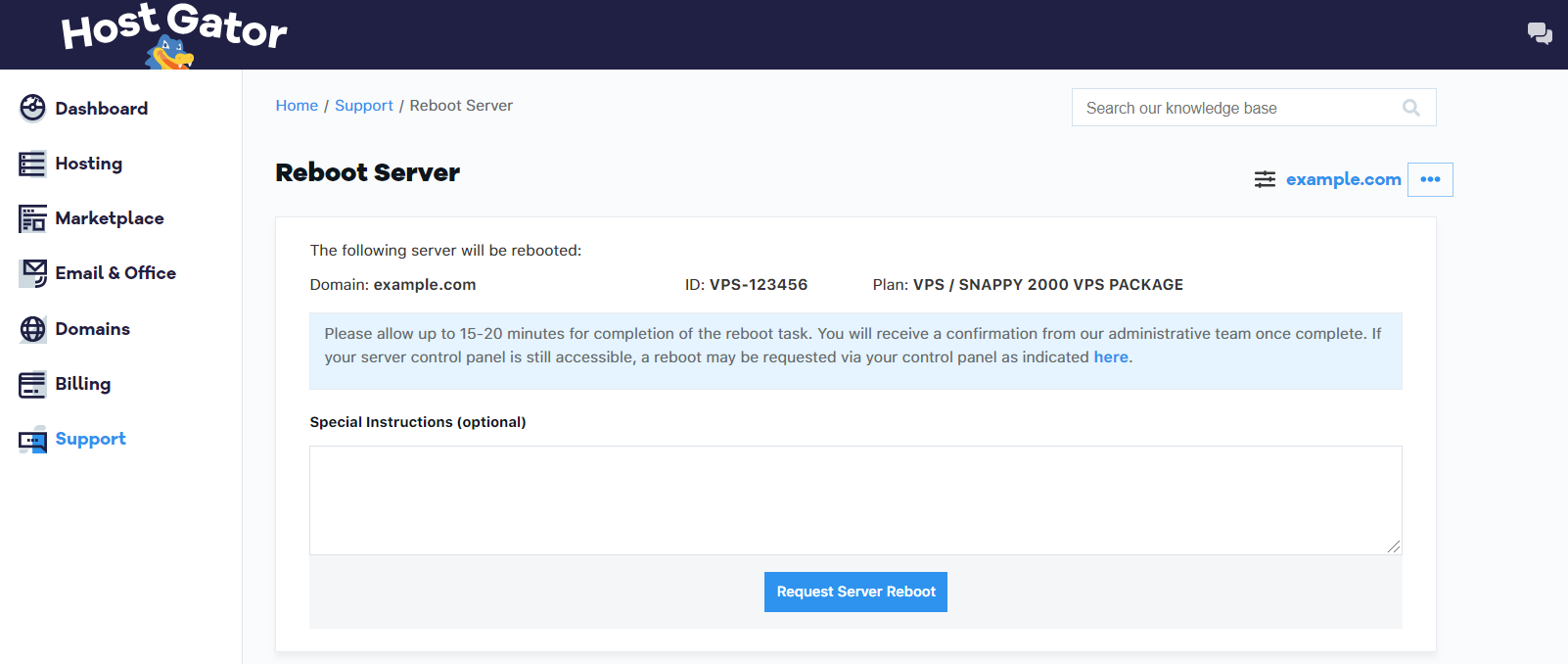A cropped screenshot of a support ticket on the HostGator website. At the top of the page, there is a prominent purple banner featuring the HostGator logo on the left and a chat box icon on the far right. A vertical navigation panel on the left side of the screen lists categories, including "Home," "Support," and "Reboot Server."

The central section of the page is headed by the title "Reboot Server" in bold black letters. Directly beneath this heading is a white text box stating, "The following server will be rebooted:" followed by "domain example.com." Adjacent to this, an ID number and a plan number are provided for reference.

Below this information, a blue banner alerts users: "Please allow up to 15-20 minutes for the completion of the reboot task. You will receive a confirmation form from our administrative team once complete. If your server control panel is still accessible, a reboot may be requested via your control panel as indicated here," with the word "here" hyperlinked.

Further down, the page includes a section labeled "Special Instructions" with "(optional)" in parentheses. Beneath this section is an empty large text box intended for any additional instructions. Centered at the bottom of the page, a prominent blue button reads "Request Server Reboot."